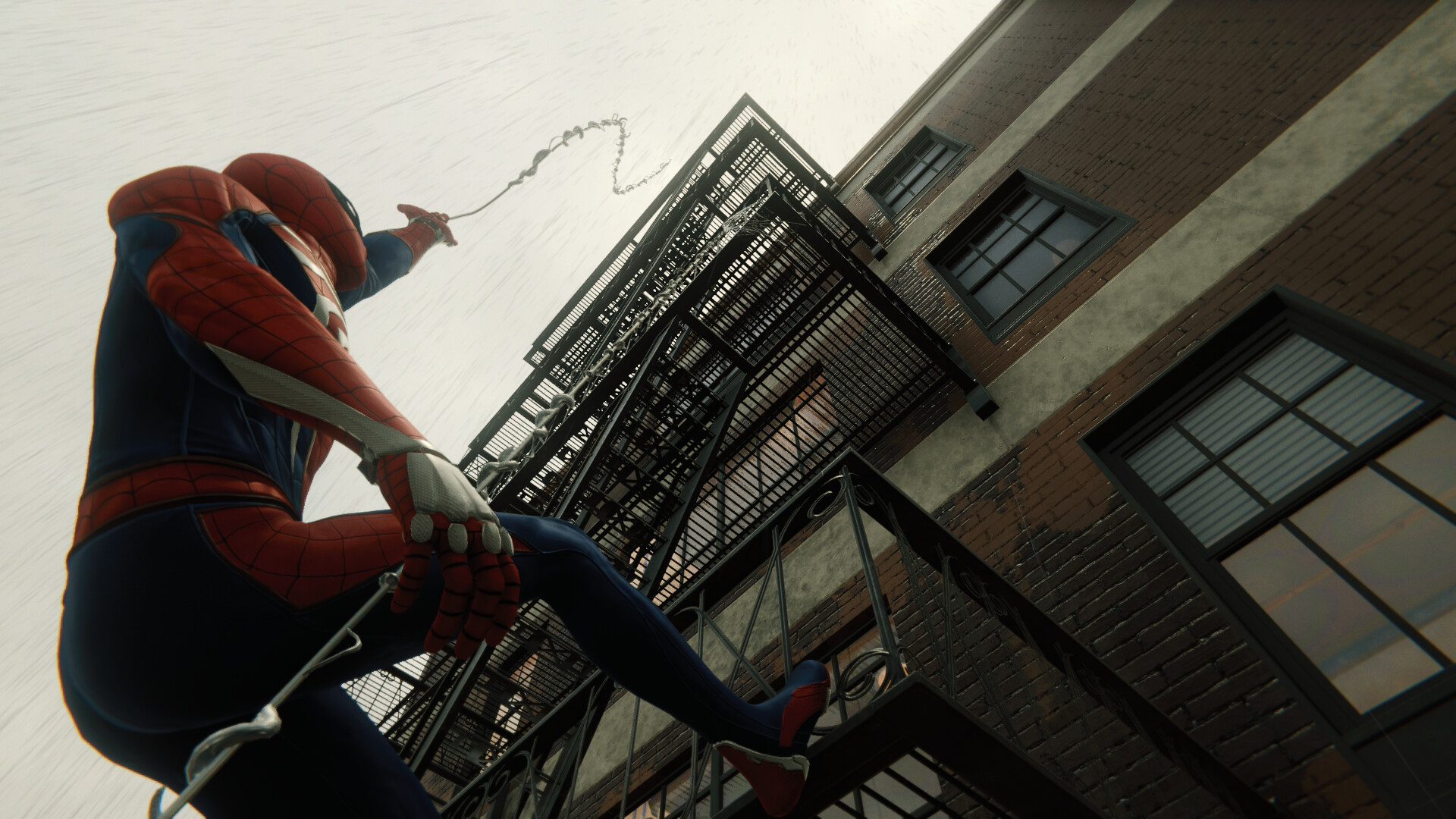This detailed image, likely computer-generated, depicts Spider-Man in his iconic red, blue, and white suit, mid-action as he shoots a web from his left hand towards the top of a fire escape attached to a red brick building. The scene is captured from a low angle, looking up, creating an impressive perspective view where Spider-Man is positioned on the left side. He has his right leg braced on the black metal steps of the fire escape while his left arm is extended, web streaming upward. The building features several black windows with white blinds, some partially open, which are separated by lines of concrete between each floor. The sky above is a light gray, typical of an overcast day, and hints of rain add to the dynamic and intense atmosphere of the scene.